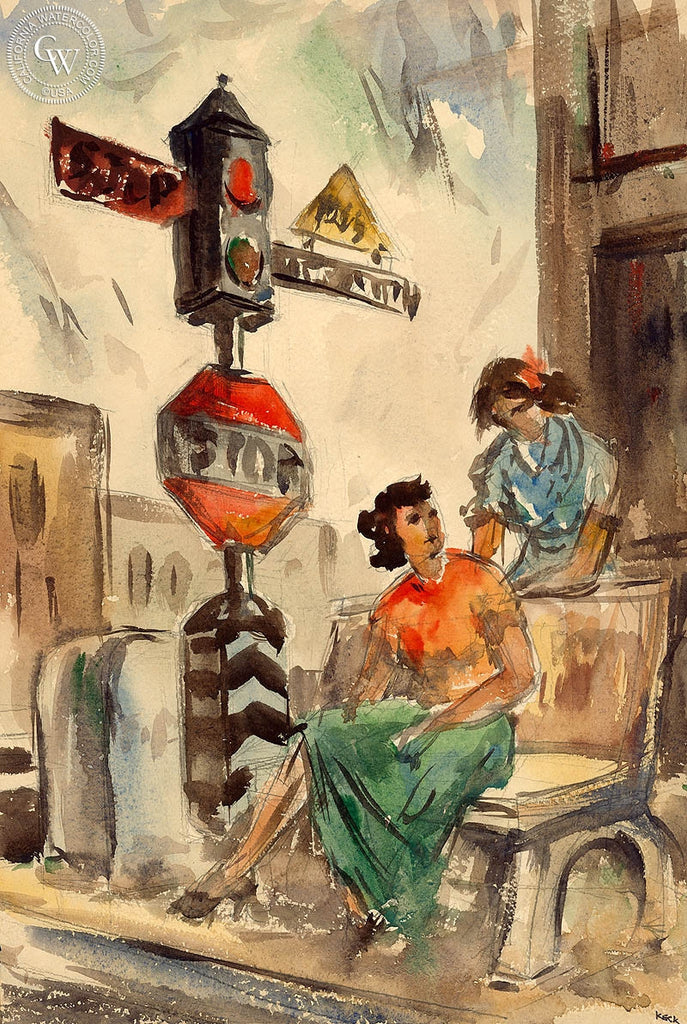This painting depicts two women at a bus stop or train stop, illustrated in a loose, sketchy style characteristic of fashion drawings, with additions of watercolour washes. The woman seated on the right is dressed in an orange top and green skirt, while the standing woman wears a blue top and has red flowers in her hair. The seated woman is on a bench that appears to be stone, and they seem engaged in conversation. Behind them, a traffic light shows a red signal, attached to a stop sign with black and white markings and a red border. The composition includes a background of buildings and sky, subtly rendered to complement the foreground figures. The top left corner of the image bears the imprint "CaliforniaWatercolor.com CW USA," confirming the medium.